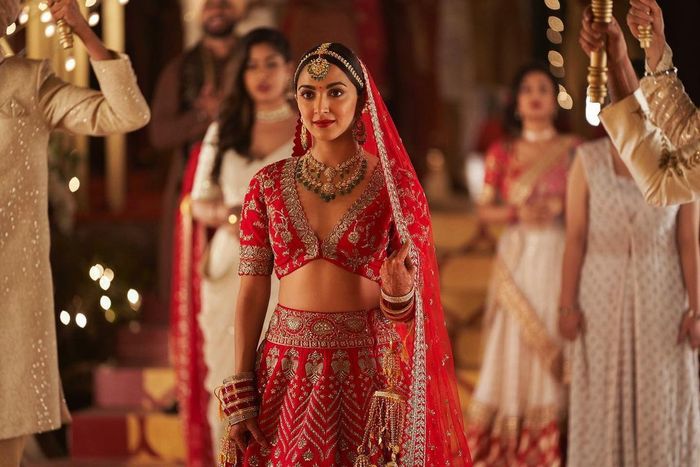The photograph captures a vibrant and ornate scene centered around a young, attractive woman of Indian or West Asian descent, likely in her late teens or early 20s, suggesting a ceremonial event, possibly a wedding. She stands out in an opulent red and white dress adorned with intricate gold embroidery, complemented by a red headscarf that drapes elegantly down her back. Her attire is embellished with numerous pieces of jewellery, including necklaces and long earrings, highlighting her cultural heritage.

She stands in the center, smiling warmly and gazing lovingly, creating a focal point in this richly decorated setting. The background reveals an ornate church-like building accented with white and coral-red decor. Flanking her are three women dressed in similarly elaborate outfits, reminiscent of a traditional bridal party formation. To the edges of the frame, there are glimpses of men dressed in cream-colored garments, possibly traditional male attire, one of whom is holding a structure or lamp above the bride's head, a detail suggesting ceremonial significance.

This stunning tableau is a vivid depiction of a cultural celebration, abundant with rich hues, intricate designs, and a palpable sense of joy and festivity.